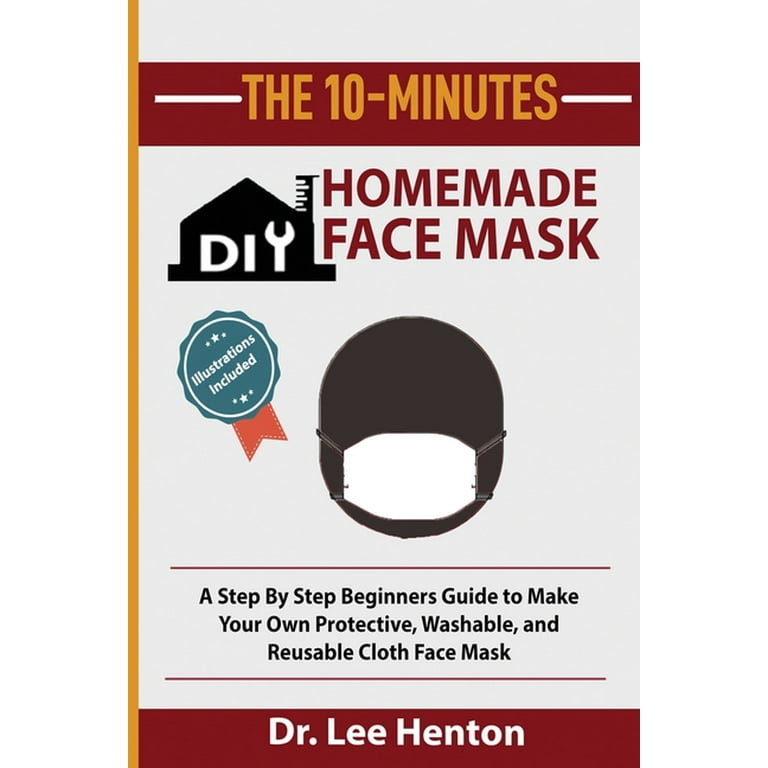The image features the cover of a book titled "The 10-Minutes DIY Homemade Face Mask." The title is prominently displayed with "10 Minutes" written in gold letters on a red banner at the top. Beneath this, the letters "DIY," with the "Y" depicted as a small wrench, are set against an illustration of a black house with a chimney. To the right, bold red text reads "Homemade Face Mask," accompanied by a simple illustration of a head wearing a white face mask. On the left side, a green ribbon with an orange tail declares "Illustrations Included." Below the illustration, text explains that it is "A Step-by-Step Beginner's Guide to Make Your Own Protective, Washable, and Reusable Cloth Face Mask." The author's name, Dr. Lee Hinton, is displayed at the bottom in white lettering on a red stripe. The spine of the book is gold, and the background of the cover is a simple white. The overall color scheme includes white, red, gold, black, green, and orange.